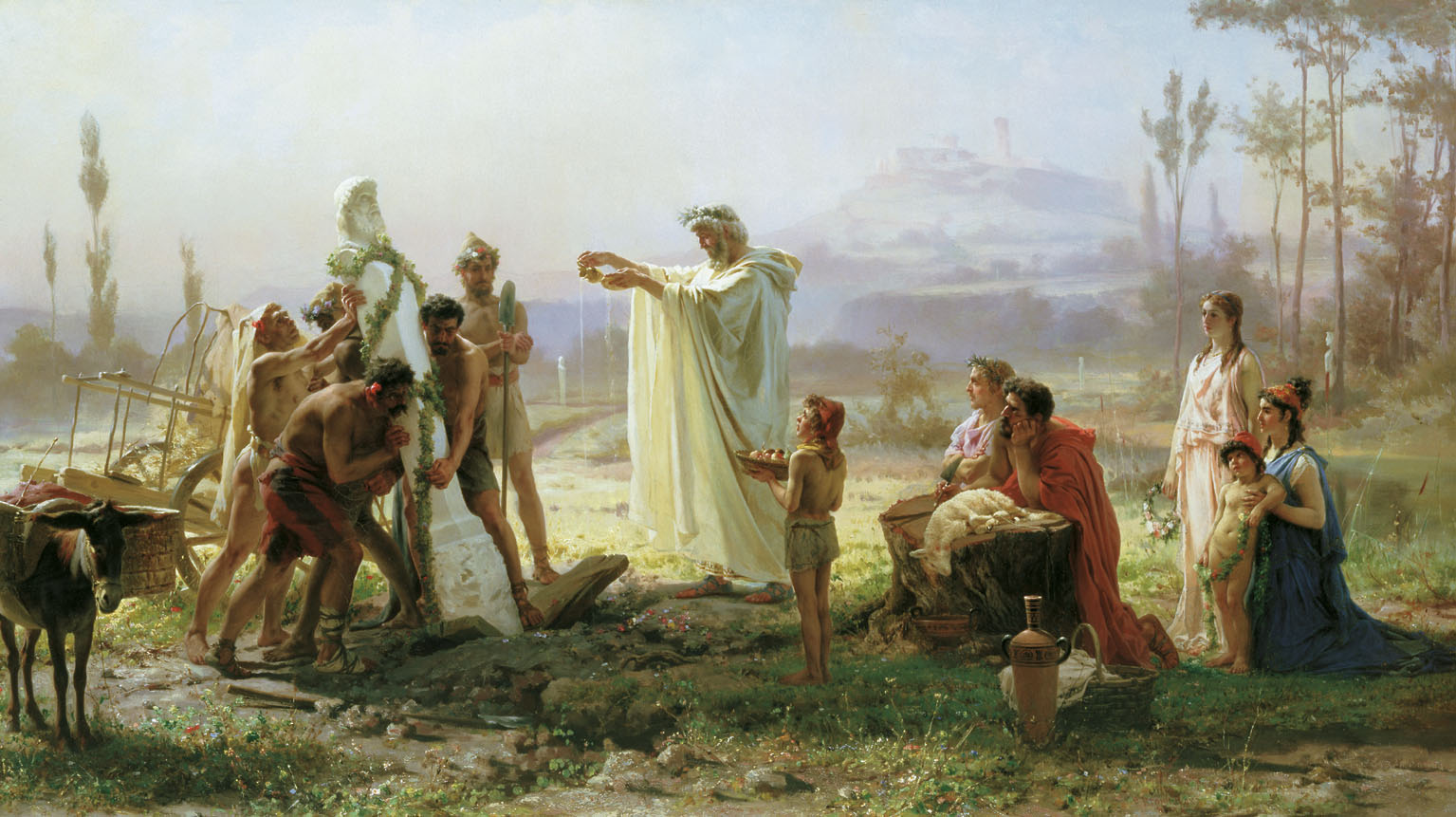In this highly detailed and realistic painting, the central figure is a white-haired and white-bearded man dressed in a long, wide robe, suggesting he's some kind of priest or saint. He extends his hands towards a scene of intense activity. To his left, four men are struggling to lift and stabilize a tall, heavy statue featuring a male bust on a pillar. Nearby, a figure who might be a Roman soldier or another authoritative figure watches over the proceedings, holding a staff. A dark brown donkey and a cart can be seen to the left, further grounding the outdoor setting.

In front of the robed man stands a little boy holding a plate of apples. A small gathering of people, comprising two men, two women, and two children, form a semi-circle behind the main action. One of the children offers a basket of fruit to the robed man. The group also includes a woman kneeling by a dead sheep positioned on a tree stump, accompanied by another woman kneeling and a child standing naked in front of her. By their side on the ground is a jug with a handle and several baskets full of various items.

The background includes lush greenery with trees and a mountain topped by a village, enhancing the serene yet solemn atmosphere. While the exact narrative remains ambiguous, the scene seems to mix elements of religious ritual, family gathering, and perhaps even burial rites, given the solemn activities and symbolic objects scattered throughout.